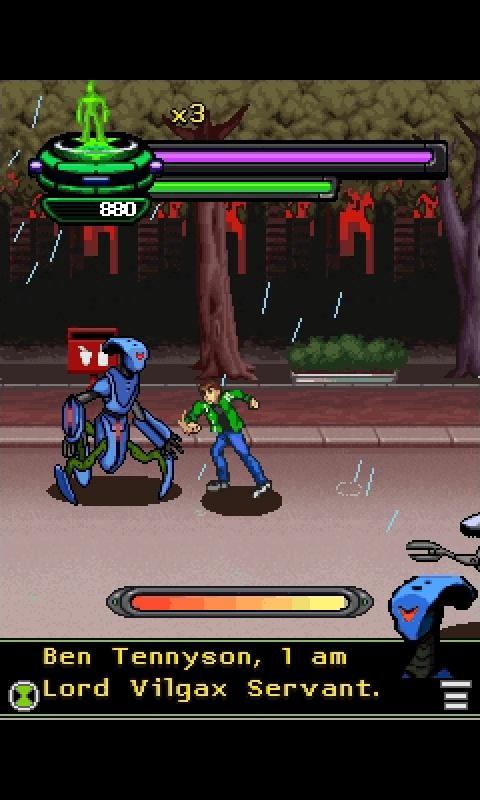This image is a screenshot from the video game "Ben 10," featuring intense confrontation between two characters. At the bottom, the text reads: "Ben Tennyson, I am Lord Vilgax's servant." The image prominently showcases two players: a young boy, presumably Ben Tennyson, wearing a green jacket and blue pants, poised to deliver a powerful punch. Opposite him stands a blue, monstrous figure with an unusual head, clad in what appears to be a coat of armor, and possessing bizarre arms and legs.

Below the characters is a progress bar that transitions in color from red to pale yellow. On the left, there's a cartoonish blue dog with a red smile, while on the right, only a silver hand of another character is visible. In the background, there is a tree adorned with red elements. At the top, two bars — one green and one purple — are displayed.

Additionally, there is a graphic depicting a flying saucer with a green figure standing on top, accompanied by the numbers "880" below and a multiplier "x3" next to it.